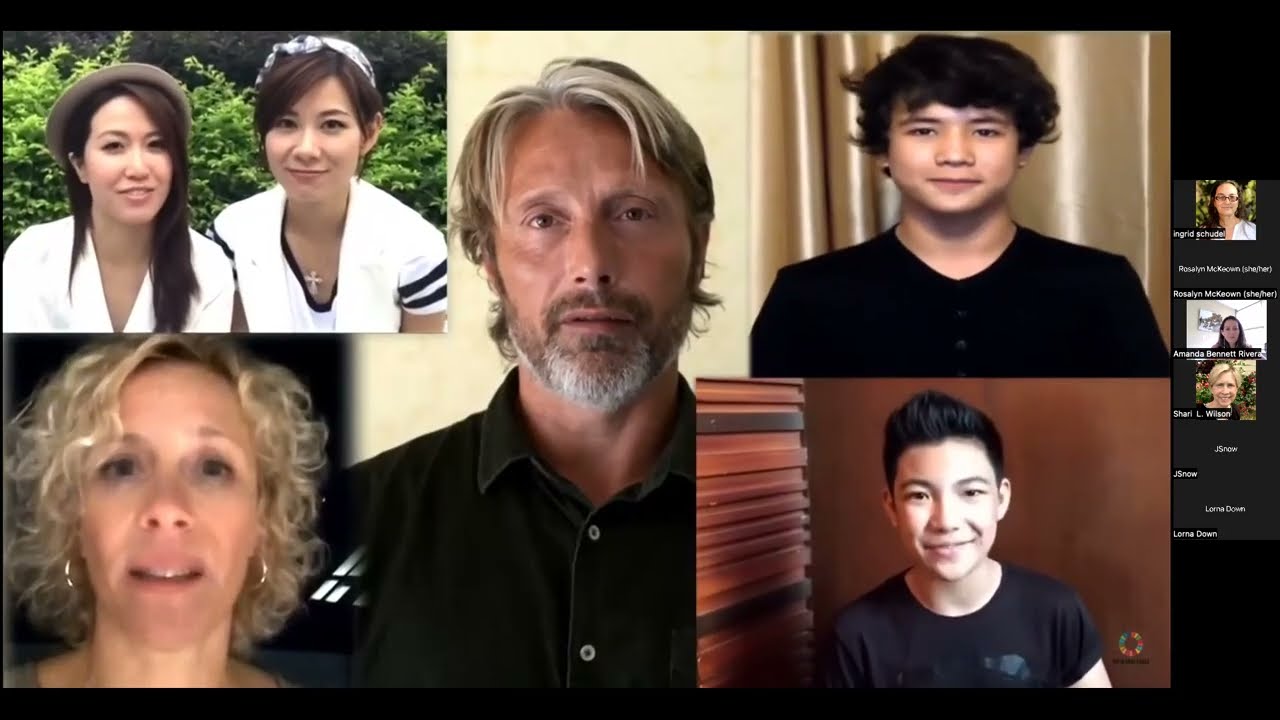This image is a detailed collage featuring six distinct individuals, each in their own separate photograph. In the top left corner, there are two Asian females who bear a striking resemblance. The female on the left is wearing a purple headband and a white shirt with two black stripes on the sleeves, while the one on the right sports a fedora hat and a white shirt with a long V-neck and a cross necklace. Below them in the bottom left corner is a white woman with short, curly blonde hair, gold hoop earrings, and a relaxed expression as she looks directly into the camera. 

At the center of the collage is an older white man, possibly in his 40s, with a salt-and-pepper goatee and similarly colored hair parted to the left, clad in a black button-down shirt. In the right upper corner is a young Asian male, likely a teenager, with shaggy black hair and a black shirt. Directly beneath him, in the bottom right corner, is another young Asian boy, slightly younger, with short spiky black hair and a black shirt, flashing a subtle smirk and standing in front of a brown doorway.